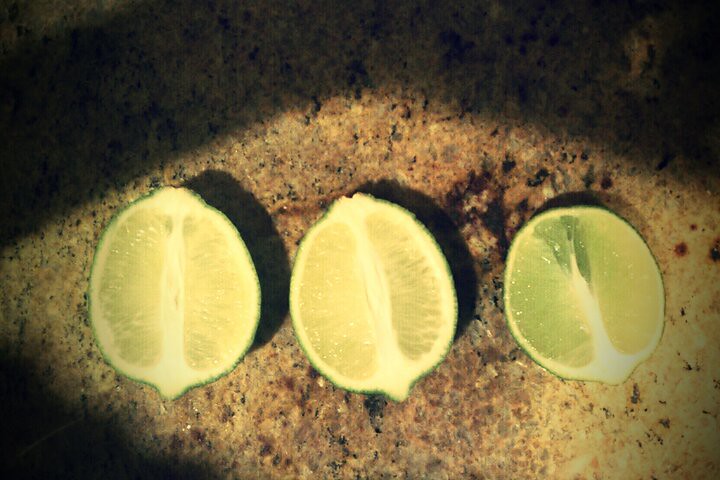This detailed close-up photo features three halved limes arranged in a row on a dark granite countertop, which has distinct brown, black, and beige spotting. The limes are positioned skin-side down, exposing their juicy, moist interiors, which are a light green-yellow color with a white rind encircling the core. The rind's darker green border contrasts with the lighter inner flesh, which is slightly translucent with visible small lines running through it. The limes are hit by an overhead diamond-shaped illumination, likely from a window or other light source, casting a shadow around them. The limes are of similar size, although the lime on the right appears a bit smaller and less perfectly formed than the other two. The lighting emphasizes the wet, fresh appearance of the limes and the intricate details of the granite countertop.